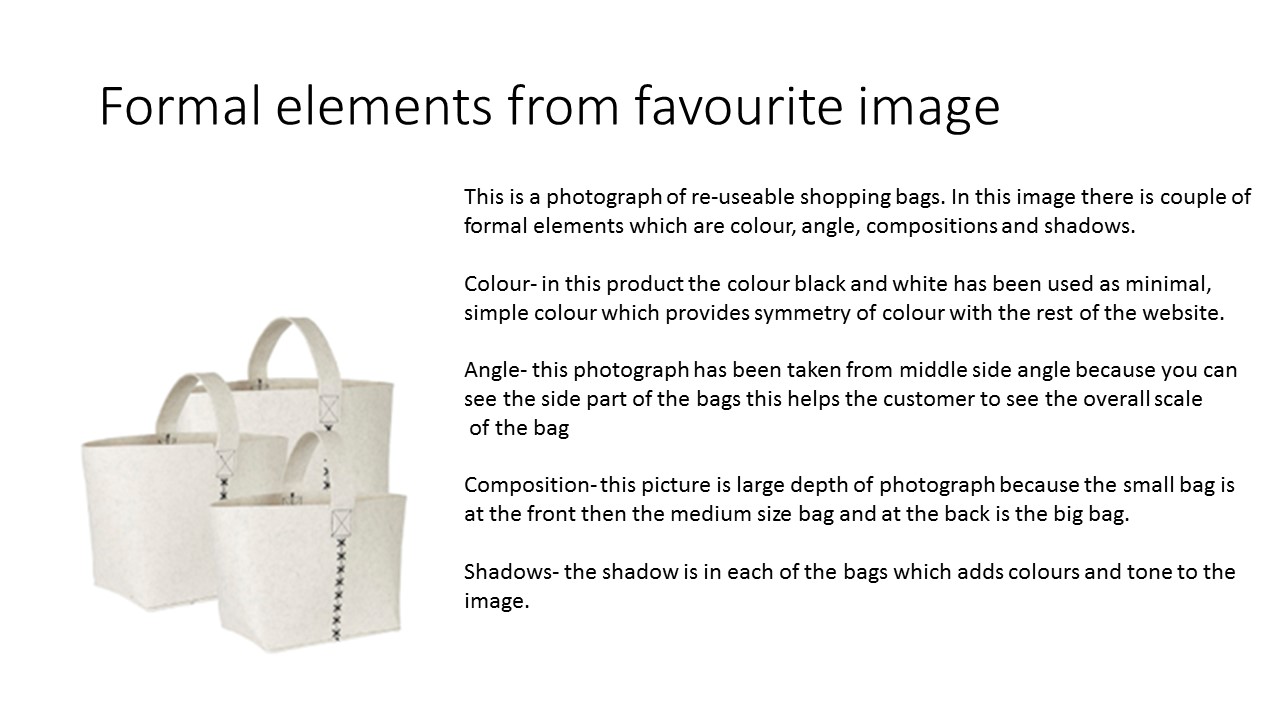This landscape image features three reusable shopping bags of varying sizes positioned on the left side, each characterized by white material with black X stitching running down the middle from the handles. The bags are arranged with the small one in the front, the medium one in the middle, and the large one in the back, creating a composition with significant depth. The photograph has been taken from a middle side angle, allowing viewers to appreciate the scale and form of each bag. The minimalist black and white color scheme of the bags echoes the symmetry of the website's design. Shadows cast by each bag add depth and tonal variation to the image. On the right side of the image, occupying approximately two-thirds, is a comprehensive description of the bags and their formal elements—color, angle, composition, and shadows. The title at the top reads "Formal Elements from Favorite Image," and all text is in black print on a white background.